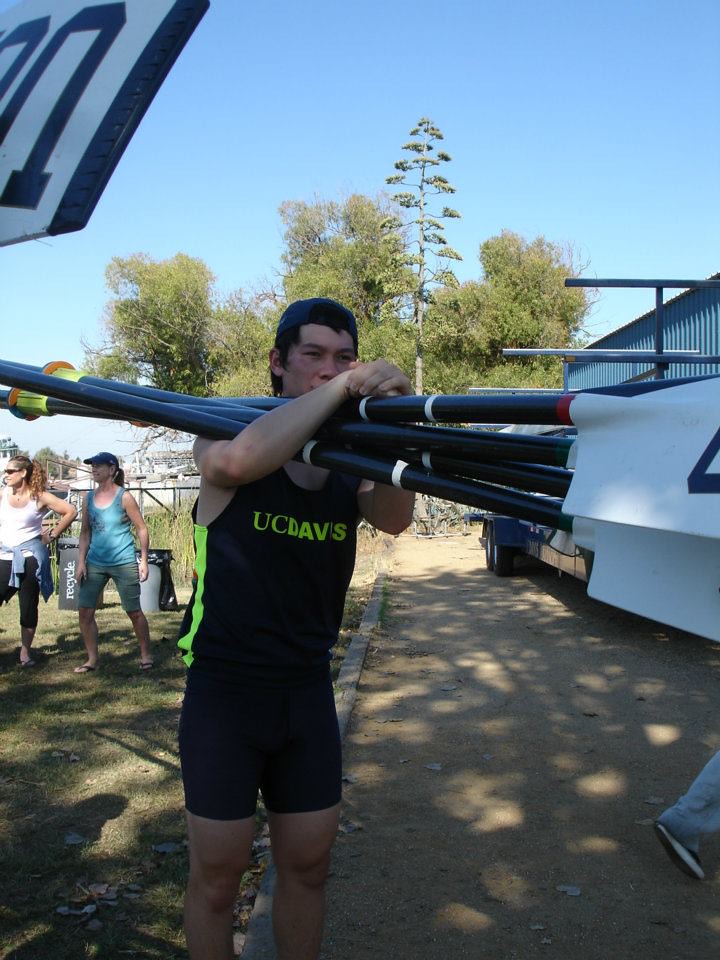This photograph captures a young man in a black tank top that says "UC Davis" in neon yellow-green lettering, and tight black shorts, likely made from a nylon-like fabric. He is wearing a baseball cap backwards and balancing approximately four boat oars over his shoulder, wrapping his arms around them for support. The oars, which have long black shafts and white paddle sections, feature orange, yellow, and possibly some numbered black lettering on their tips. The scene is set on a sunny day with a clear blue sky, framed by abundant trees and a body of water visible in the background. Nearby, a couple of women are standing and looking to their right. The man appears to be walking along a sidewalk towards a large parked truck, and there is another person visible only from the knees down, walking ahead of him.